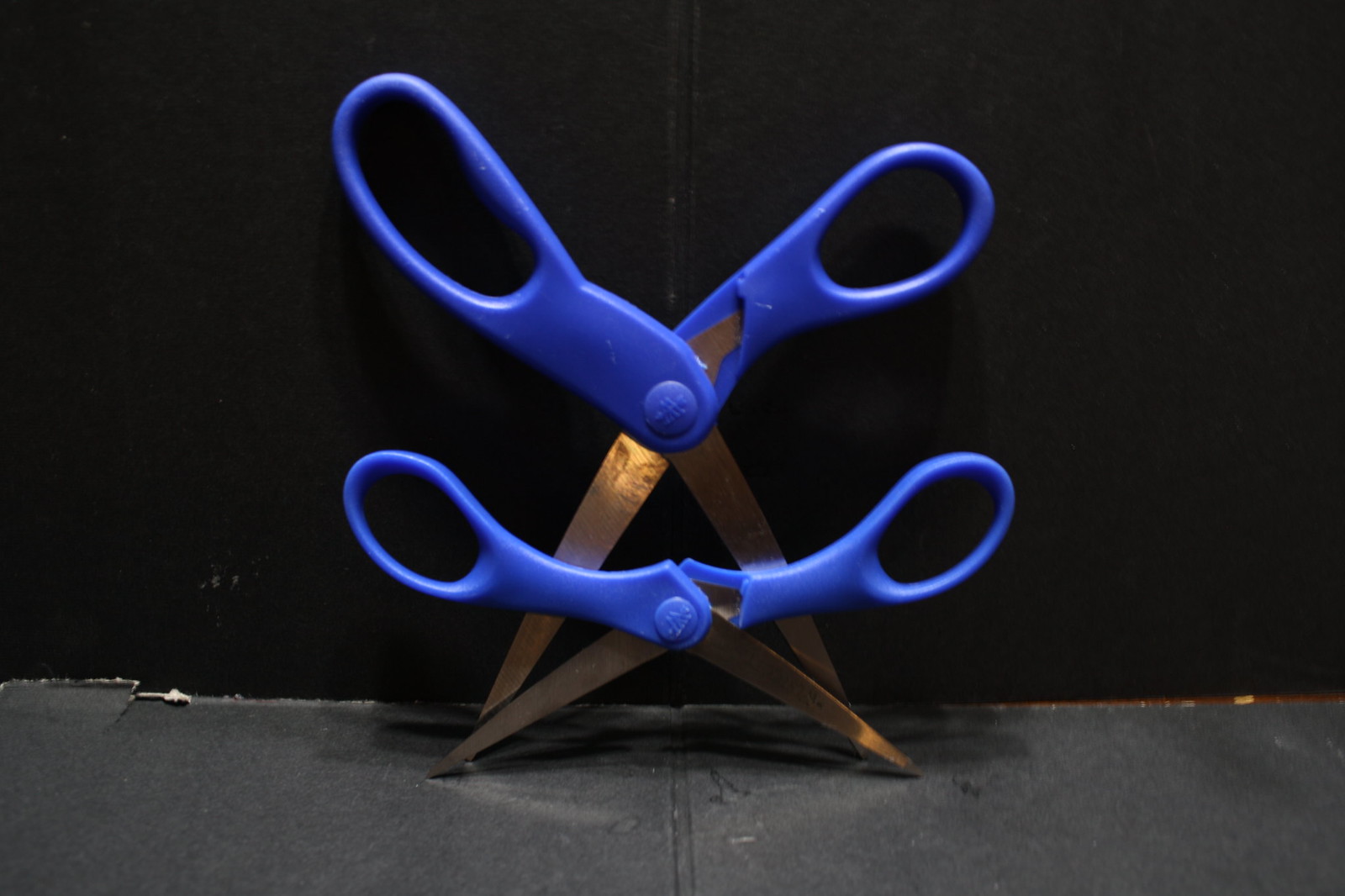In this photograph, two pairs of scissors with bright blue handles are standing upright on their blades, which are open wide to support their stance. The larger pair stands behind the smaller pair, both leaning against a black wall with a visible crease running vertically down the middle. The scissors' blades, made of silvery metal with some dark markings of wear, contrast against the gray sub-material they rest on. The background, though mainly black, has a slight separation from the floor, revealing some brown material in between, creating an imperfect connection. The larger pair features bulk covers over the screw area, and both pairs display a rusty appearance on their blades. This arrangement may serve as an artistic composition, marked by the juxtaposition of their sizes and the worn texture of the blades against the stark, slightly dirty black and gray setting.